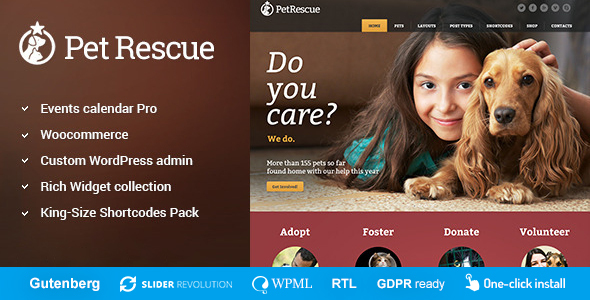This image features a detailed screenshot against a brown background themed around pet rescue. At the top, there is a circle with an illustration of a dog adorned with a star on its head. The screenshot also includes a list with check marks in front of each item: Events, Calendar Pro, WooCommerce, Custom WordPress, Admin, Rich Widget Collection, King Size, Shortcodes Pack.

In the center of the image, there is a heartfelt photograph of a girl with a dog, complemented by the text, "Do you care? We do," in a mix of vibrant yellow and white fonts. Beneath this, a message highlights the success of the platform, stating, "More than 155 pets found their homes with our help this year."

Toward the lower section, there are four distinct circles each with a call-to-action label: Adopt, Foster, Donate, and Volunteer. At the very bottom, a blue rectangle with the text "Gutenberg" is displayed, featuring a refresh symbol adjacent to it. Additional features listed include: Slider Revolution (with "Slider" in bold), WPML, RTL, GDPR Ready, and One-Click Install.